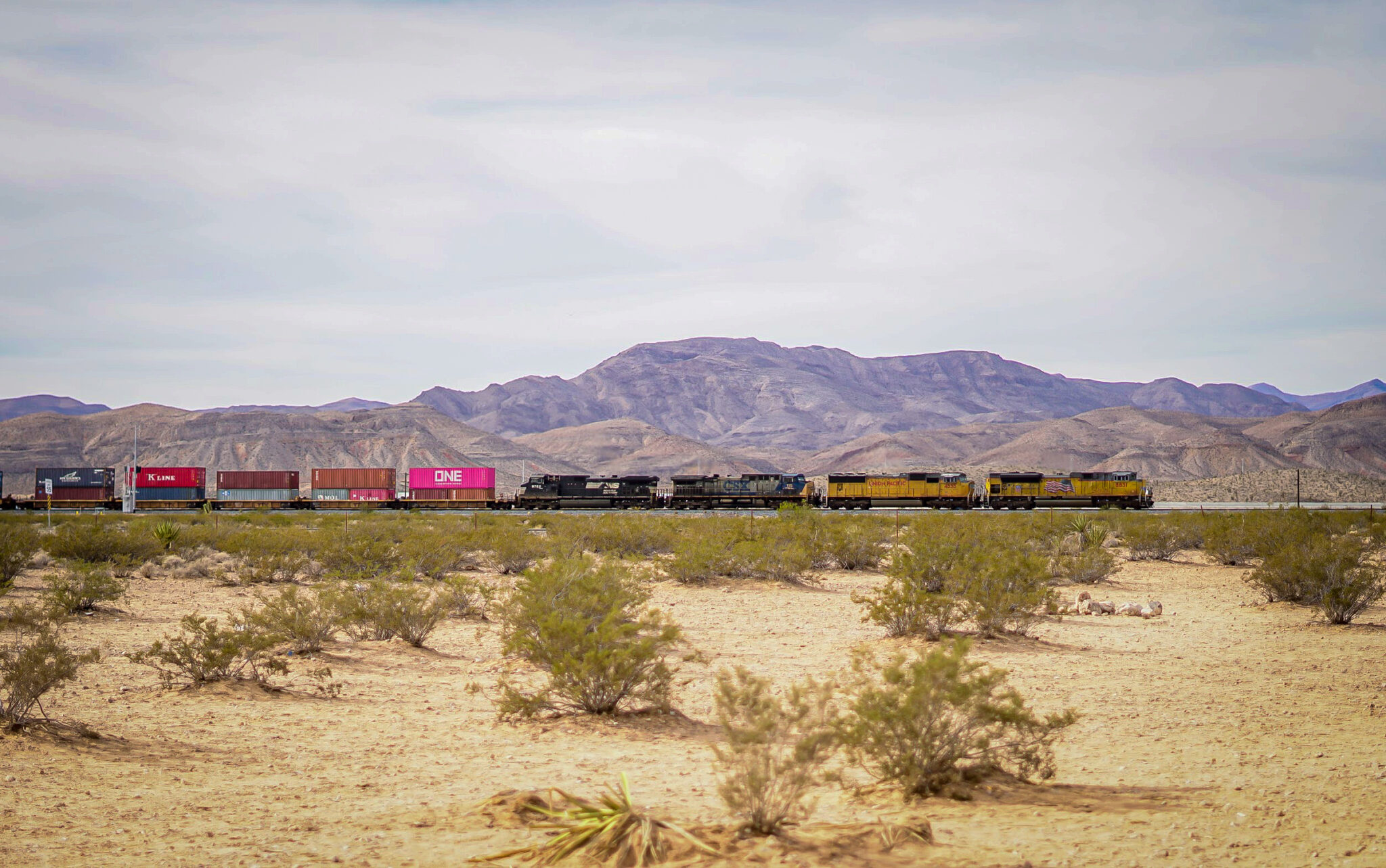In this detailed landscape photograph taken outdoors, a train travels through a sandy desert terrain adorned with sparse low-growing green shrubs. Dominating the scene is a mountain range with rocky, barren peaks and minimal vegetation. The sky above is a subdued mix of light white clouds with occasional patches of blue. The train, which heads towards the right side of the image, features a series of distinct cars: starting with a yellow main engine, followed by another yellow car, a blue car labeled "CSK," a black car with markings, and an assortment of about ten cargo containers in various colors. Notable among them are a red container marked "Kwan" and several others loaded onto flatbed platforms. The setting evokes a stark, yet picturesque desert environment with the train providing a striking contrast as it traverses the central train tracks splitting the photograph.